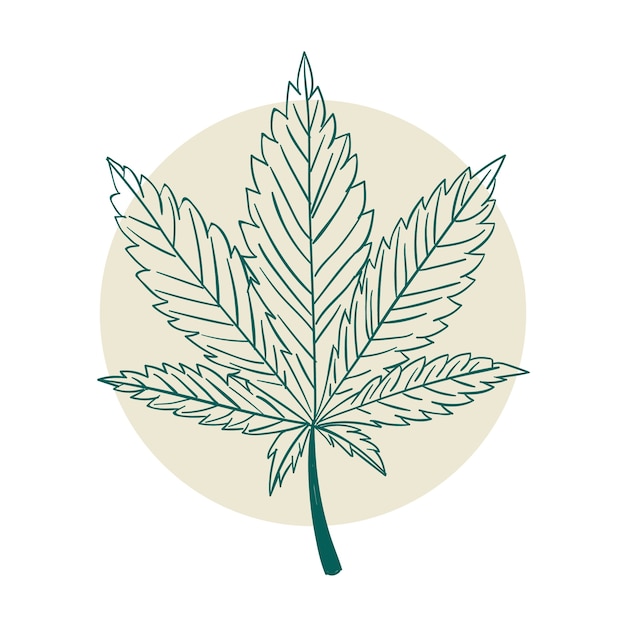The image illustrates a detailed and somewhat symmetrical maple leaf with five main frayed sections, highlighted by dark green outlines. The leaf, uncolored and presented purely through line art, slightly overflows a central, very light green (almost beige) circle that serves as the background. The stem of the leaf is fully shaded in dark green, creating a bold contrast against the light, almost transparent circle backdrop. The minimalist design focuses on the primary structures of the leaf, emphasizing its intricate and characteristic shape.